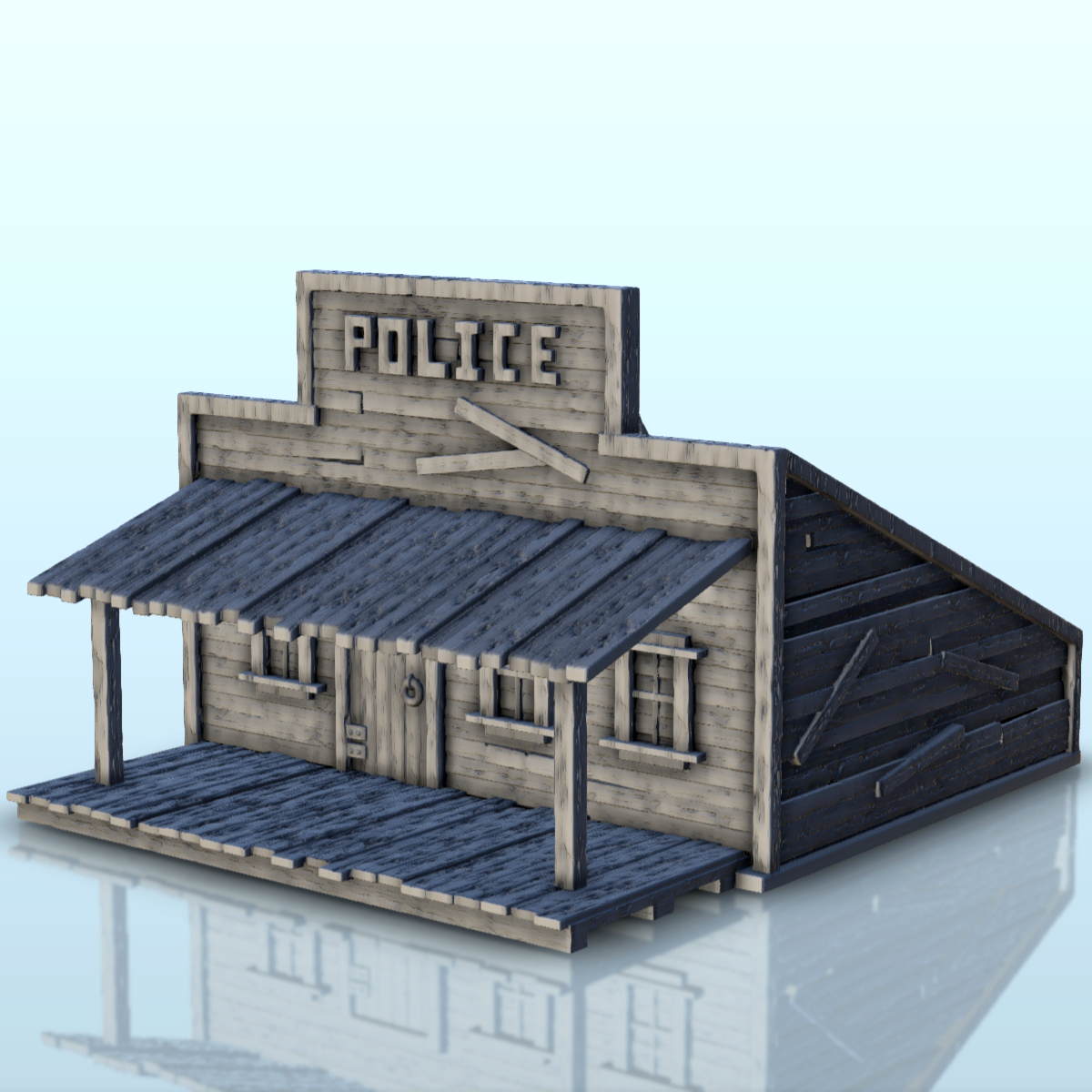The image displays a 3D digital rendering of a small, weathered wooden building, likely a police station, with an overall triangular shape. The building stands on a light blue, reflective surface. The structure features a sloping roof, with the back roofline tapering down sharply, and a flat front facade. Above the main entrance, which includes a door and three windows, there is a large sign crafted from the same aged wood as the building, spelling out "POLICE." The entrance is accentuated by a small covered porch supported by beams at each end. The weathered appearance and simplistic design suggest a rustic, old-fashioned style, apt for a digital asset in a video game. The side walls predominantly consist of grayish, wooden planks, with additional planks attached to give the building an even more outdated and unrefined look.